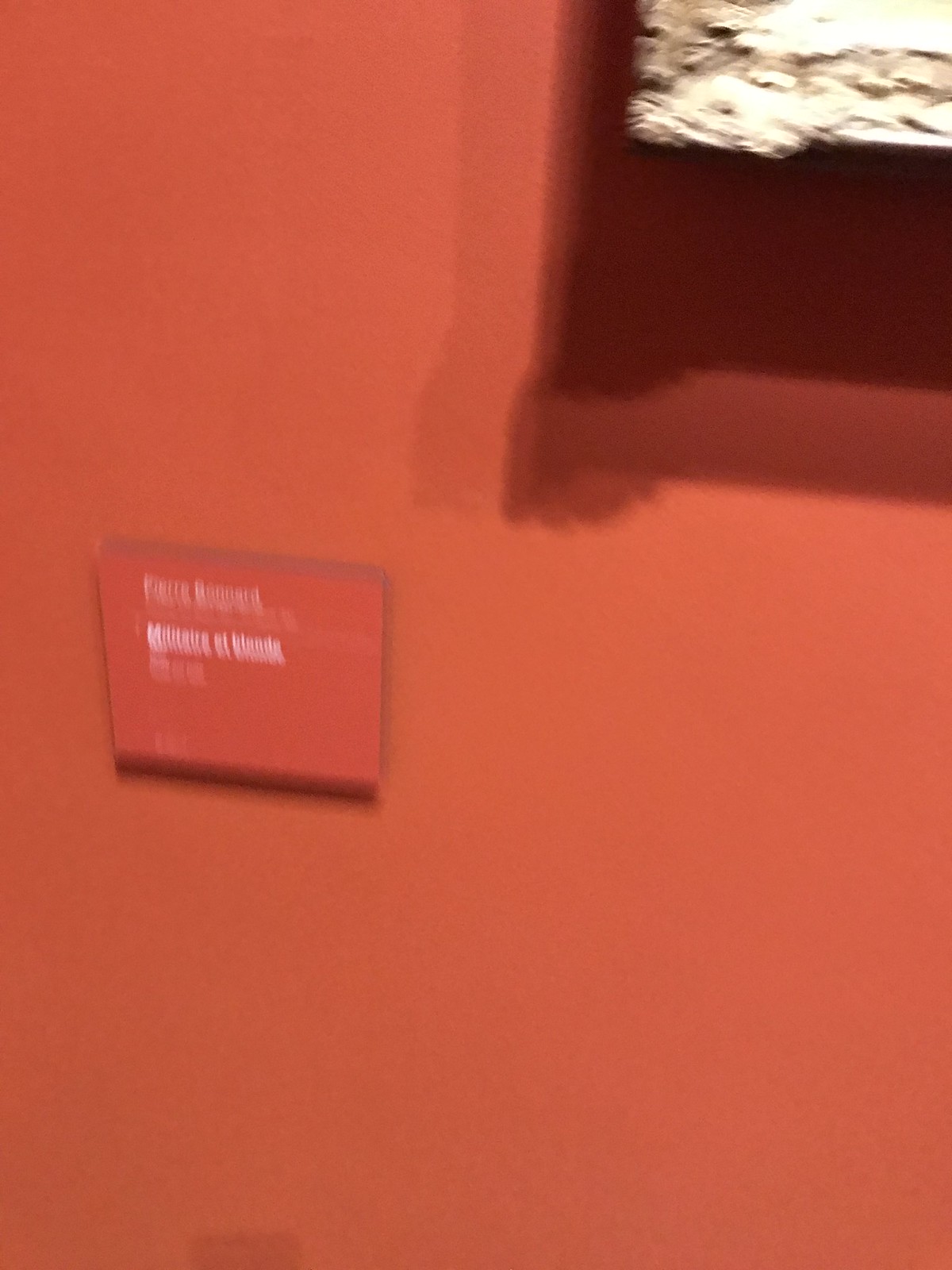This rectangular, vertically-oriented color photograph predominantly features a deep red hue, though the entire scene is significantly out of focus, lending an impressionistic quality to the image. The blurred effect makes it difficult to discern fine details, creating a sense that the photo might be capturing an exhibit wall in a museum. In the mid-left portion of the image, there appears to be a small object affixed to the wall, also a shade of red but slightly darker. This object has white lettering, though the blur obscures the ability to read the text. In the upper right corner, the faint outline of what might be a square or another display element is barely visible, casting subtle shadows below it. The overall atmosphere is one of indistinct shapes and shadows, contributing to a mysterious and abstract aesthetic.